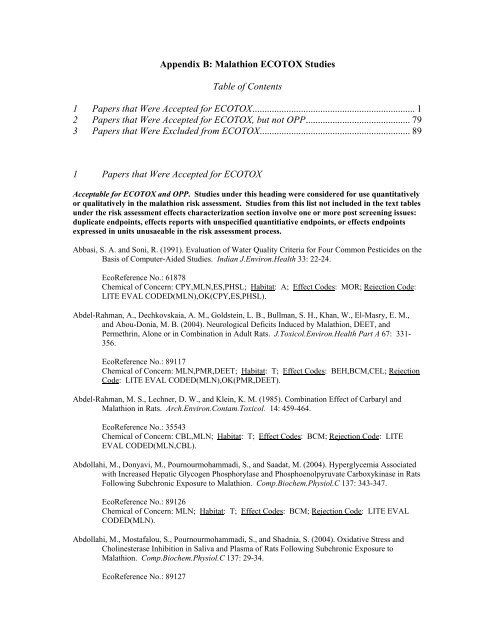This image is a page from a book detailing the Appendix B of the Malathion Ecotox Studies. The text is primarily black, with some sections in bold. At the top, "Appendix B: Malathion Ecotox Studies" is clearly stated, followed by a centered "Table of Contents." Three main parts are listed: 

1. "Papers that were accepted for Ecotox," indicating page 1.
2. "Papers that were accepted for Ecotox but not OPP."
3. "Papers that were excluded from Ecotox," indicating page 89.

Beneath the table of contents, there is a bold paragraph titled "Acceptable for Ecotox and OPP," which explains that studies under this heading were considered for use either quantitatively or qualitatively in the Malathion risk assessment. It details criteria such as duplicate endpoints and reports with unspecified quantitative endpoints, or those expressed in units unusable in the risk assessment process. Additionally, five references are cited, with the last one noted as reference number 89127. The overall presentation consists of structured text on a white background, providing a comprehensive overview of the studies included and excluded in the Malathion Ecotox analysis.